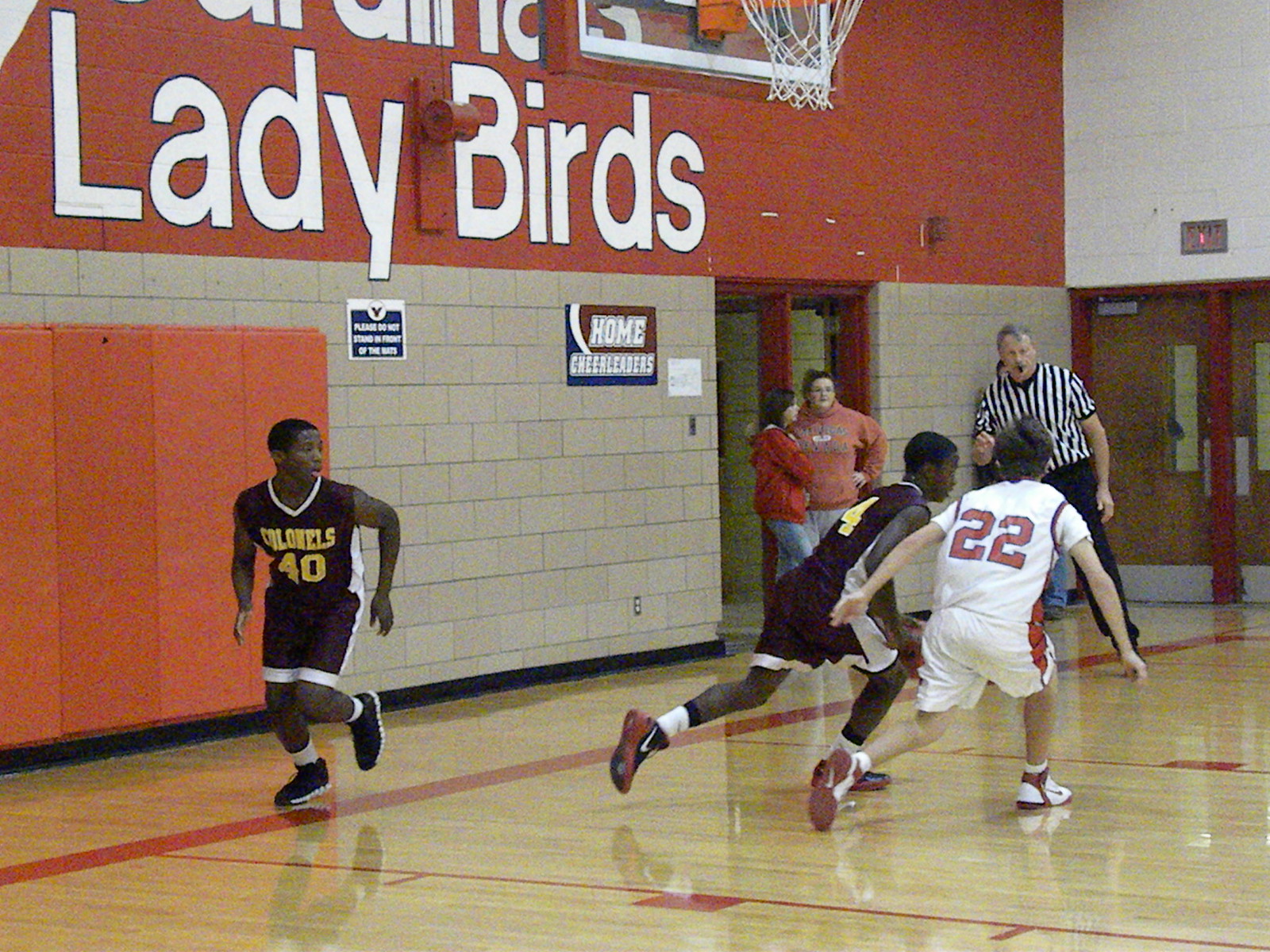This image captures an intense moment during an indoor high school basketball game on a light brown court with red markings. The scene is set against a backdrop featuring a red brick wall with the words "Lady Birds" prominently displayed in large white letters. Three players are visible: two are black boys wearing maroon-colored jerseys inscribed with "Colonels." One of them, number 40, appears to be running out of bounds on the left side of the frame, while the other, number 4, is leaning over, actively dribbling the ball. They are being guarded by a white boy wearing a white jersey with a red number 22, his black hair tied back, and sporting white and red Air Jordans. A referee dressed in black trousers and a black-and-white striped shirt is seen in the background, whistle in mouth, closely monitoring the action. Additionally, there are two women standing and conversing by a doorway, further adding to the vibrancy of the scene. The colors in the picture include shades of white, brown, orange, beige, black, oxblood, and accents of red and gold.